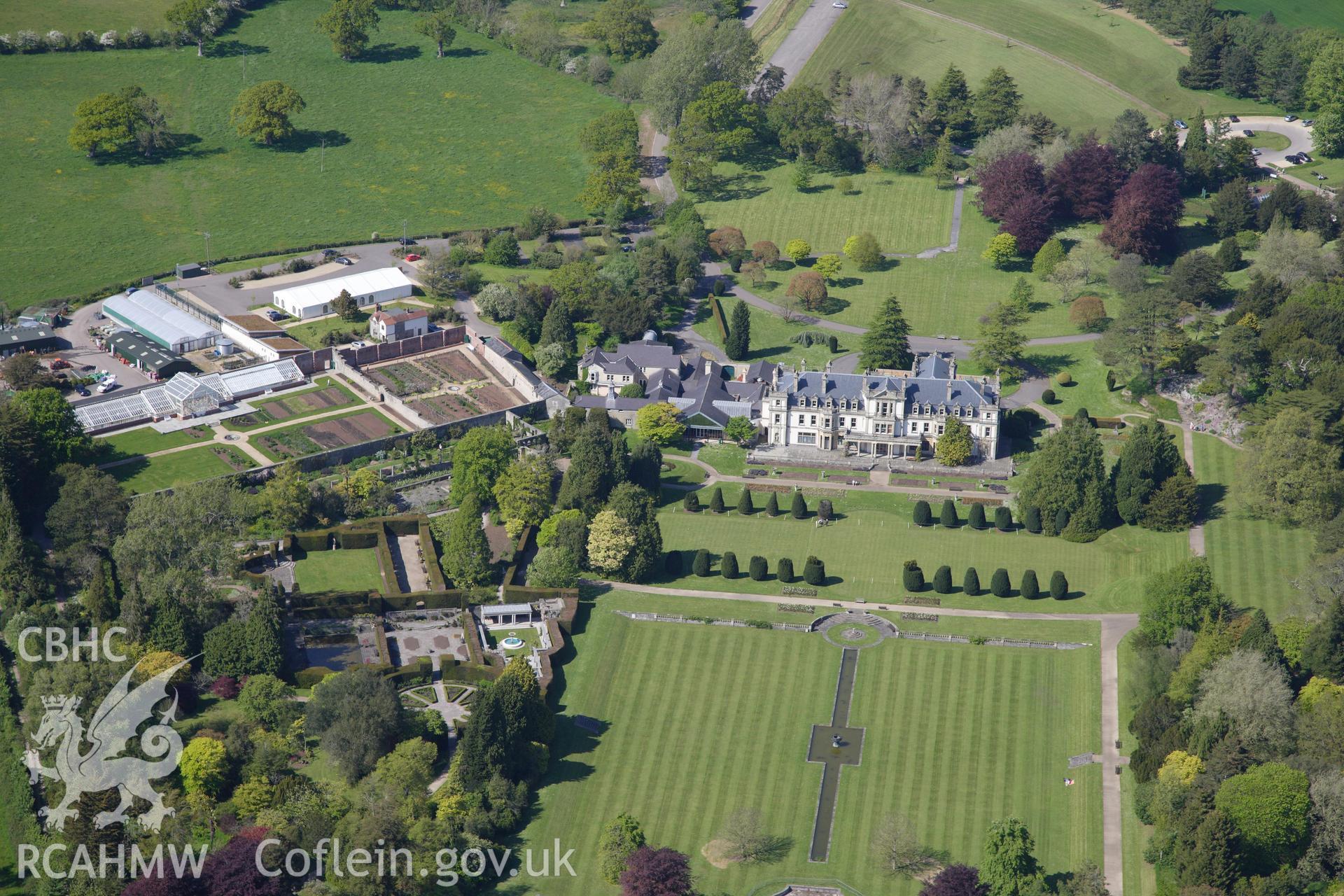This is an aerial photograph, likely taken from a plane or helicopter, showcasing a sprawling estate with meticulously landscaped grounds. The lower portion of the image reveals a striking pattern of light and dark green grass, neatly cut into alternating lines. In the center of this area sits a cement section, featuring a long rectangular walkway flanked by a smaller, thicker rectangle, likely housing a fountain amid landscaped greenery. Surrounding this central area, the right and left sides are bordered by varied trees showcasing green, yellow, and gray leaves. 

Moving up, the scene transitions to a second section adorned with green bushes outlining a slender rectangular patch of grass. Dominating the middle of the photograph stands a grand white mansion with a gray roof, exhibiting numerous windows. Beyond the mansion, additional expanses of well-manicured grass and a diverse array of trees—including some with purple and gray leaves—stretch into the distance, adding layers of depth and richness to the view.

Notable details include a white dragon emblem in the lower left-hand corner with the text “RCAHMWCOFLEIN.GOV.UK.” Further back in the image, various paths and gardens weave through the landscape, emphasizing the estate’s grandeur and the extensive planning that has gone into its design. The overall palette is predominantly green with touches of white, accentuated by earthy tones of brown and yellow, capturing the lush and serene atmosphere of the daytime setting.